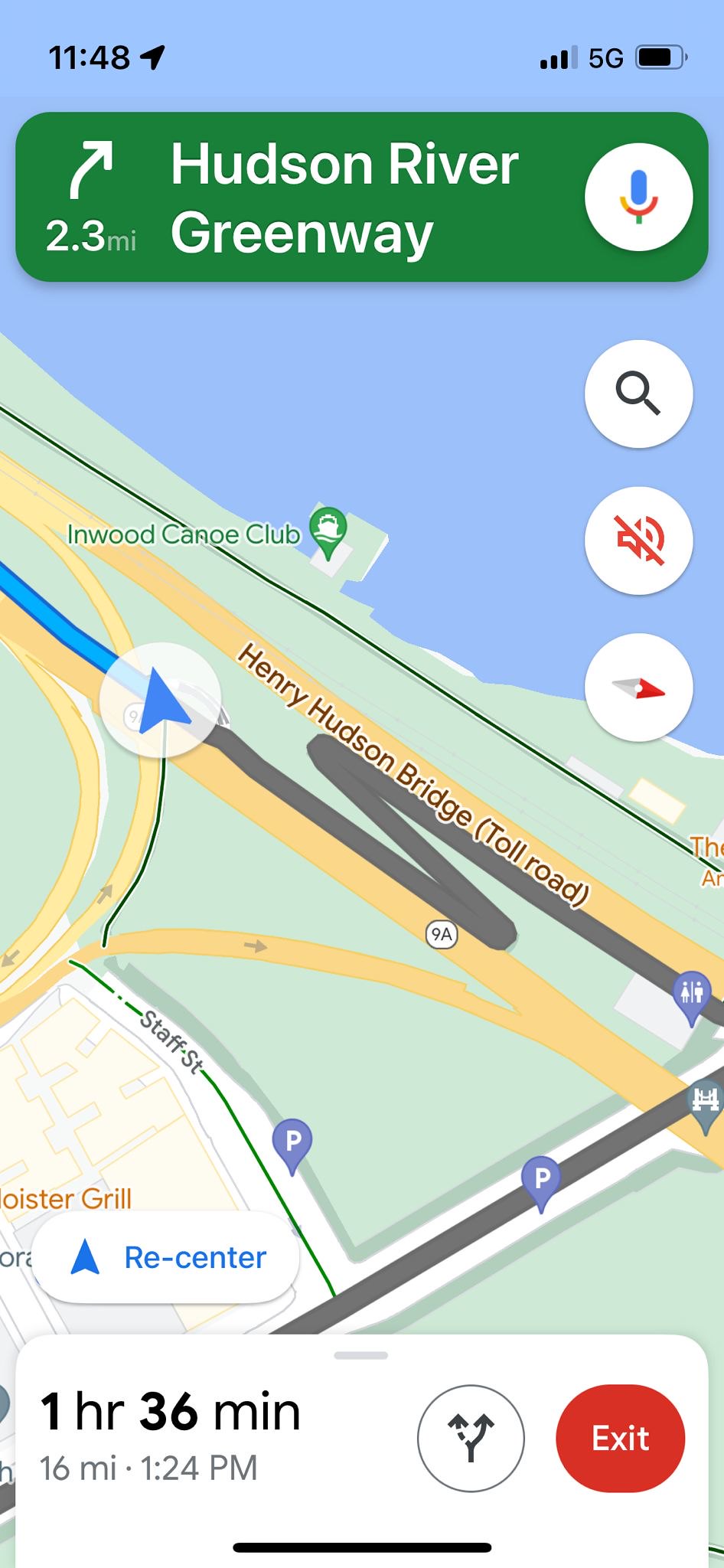The image is a detailed screenshot from a smartphone displaying the Google Maps interface. At the top of the screen, the status bar shows the time as 11:48, signal bars, a 5G indicator, and a battery icon. Below this, there is a green section with a right arrow indicating an upcoming turn in 2.3 miles for the Hudson River Greenway. The map itself prominently features a zoomed-in view of the Harry Hudson Bridge and surrounding intersecting streets, with a blue arrow representing the current position. A waterbody is visible alongside the bridge. At the bottom of the screen, the interface details that there is 1 hour and 36 minutes remaining for a 16-mile journey, with additional options like route change, recenter, and an exit button also visible on the interface.